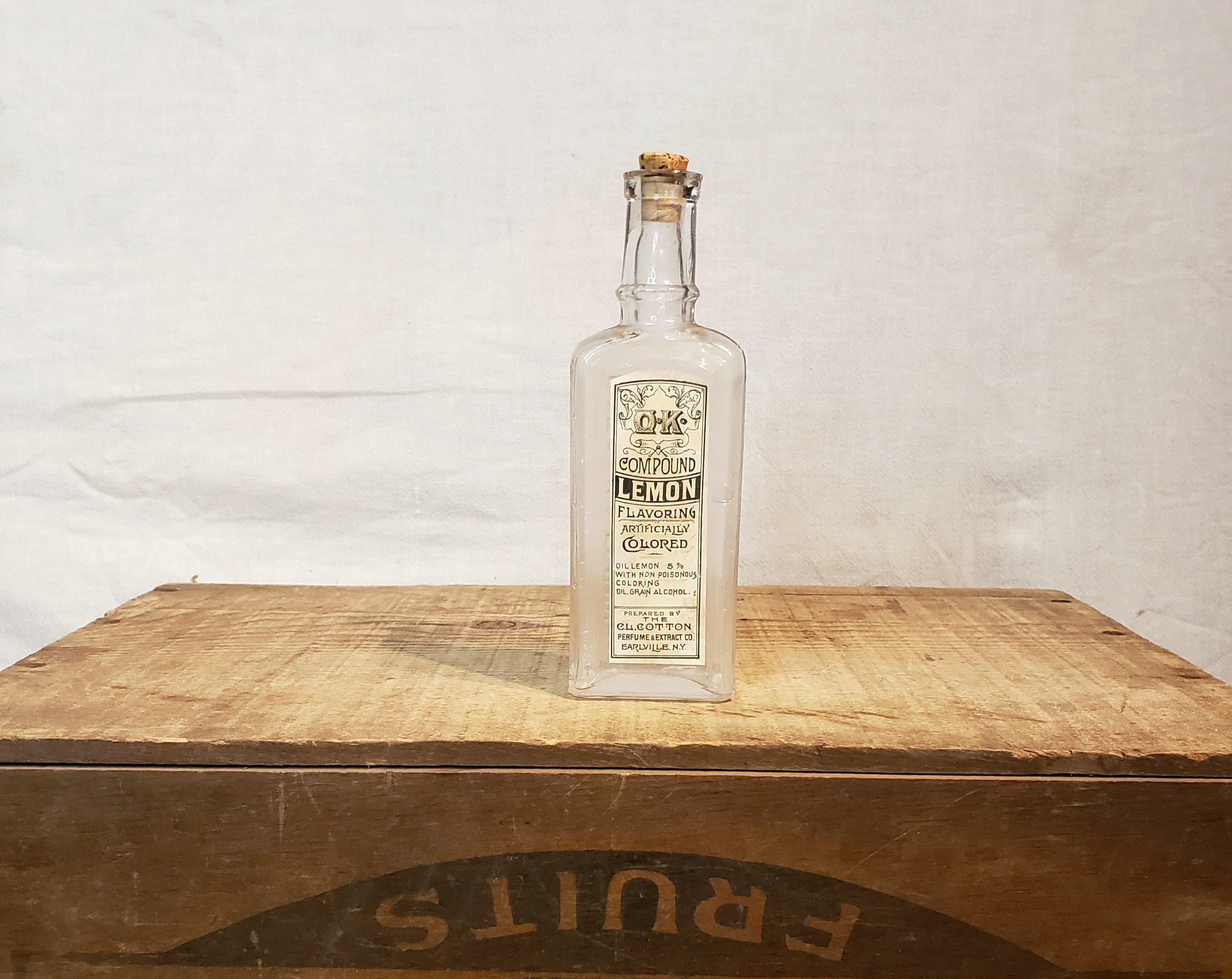This color photograph captures a vintage clear glass bottle prominently positioned on a rustic wooden crate against a white wall backdrop. The bottle, which features a tan cork at its top, boasts a white label with black ink that reads, "OK Compound Lemon Flavoring, Artificially Colored." Below this primary text, there are additional blue inscriptions detailing the ingredients and manufacturer, though they are too small to decipher. The wooden crate has a thin lid, and its rough texture underscores its age. Notably, at the bottom front of the crate, the word "fruits" is stamped in a black circle, displayed upside down. The label and the antique design of both the bottle and the crate suggest a product from the 1920s or earlier, adding to the photograph's nostalgic aura.